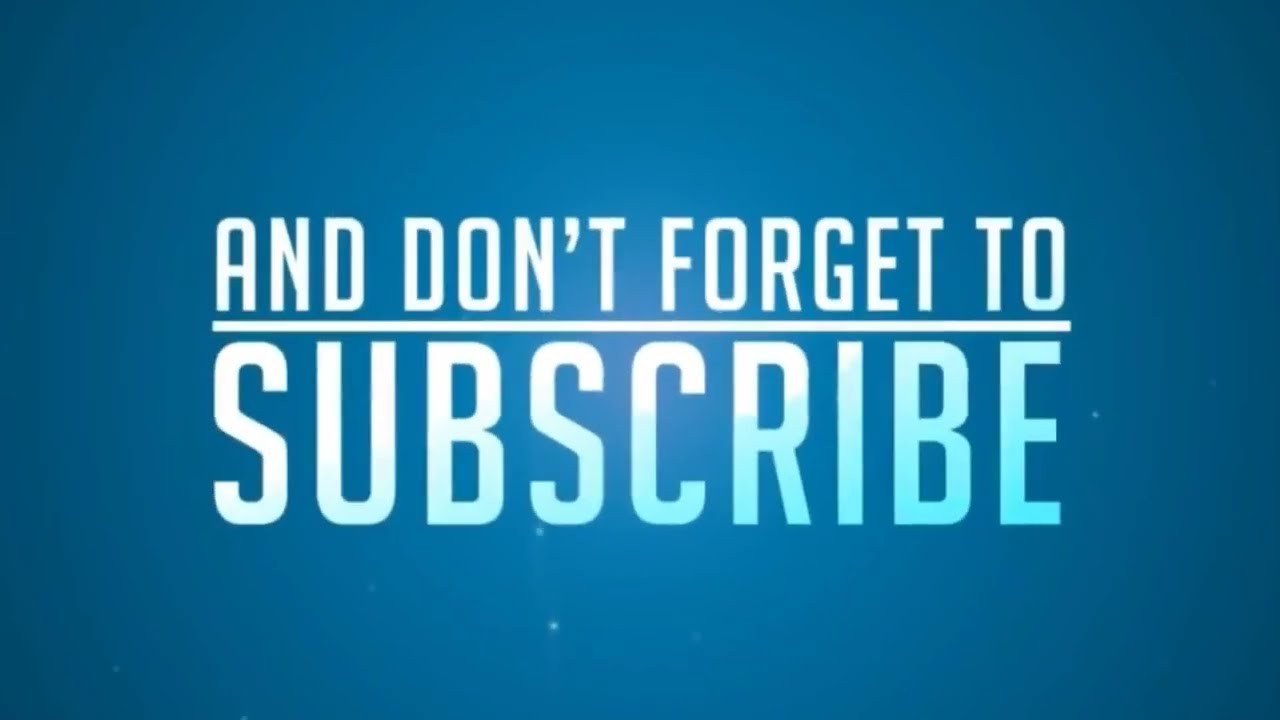The image features a rectangular flyer or advertisement with a gradient blue background that transitions from darker shades at the edges to a lighter blue in the center. The text is prominently placed with center and middle justification. At the top, a larger white underlined text states "AND DON'T FORGET TO," with the underline spanning the entire length of the phrase. Below this, the word "SUBSCRIBE" is written in an even larger font. The text "SUBSCRIBE" begins in white at the top left, gradually transforming into a light aqua blue towards the bottom right. The background is subtly decorated with tiny white speckles, resembling a starry sky.